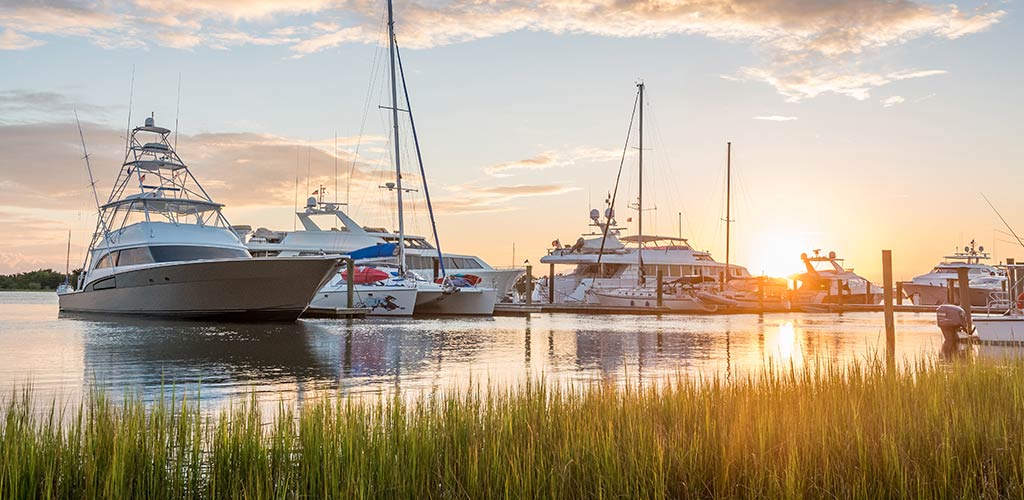This image captures a serene boat marina at either dusk or sunrise. The sky occupies about half of the image, transitioning from a whitish blue to a warm golden hue near the horizon, where the sun is positioned on the left third. Puffy white clouds are scattered in the sky. The bottom half features a water scene with tall marsh grass emerging from the foreground, leading into a stretch of water populated by at least six large boats, one of which has partially obscured artwork on its side. The boats vary in type, including party boats, catamarans, and what appears to be a sailboat in the distance. Made of metal, these vessels have various extensions rising from their centers. On the far left, a person can be seen wading in the water near one of the boats, adding a human touch to this tranquil scene.